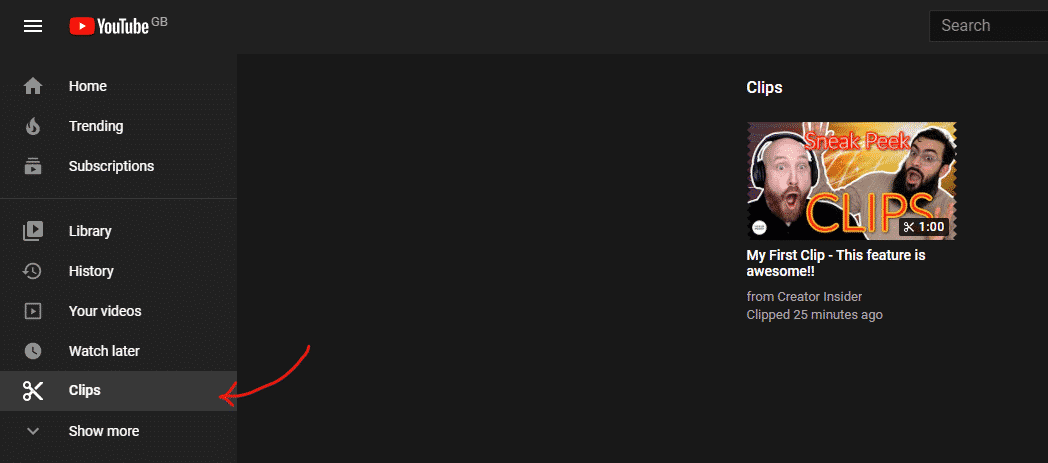This image is a screenshot of the YouTube interface in dark mode, likely taken from a desktop or web app version of the platform. The color scheme features a dark, almost black background contrasted by a gray header at the top and a gray column on the left-hand side. 

At the top left of the interface in the gray header, there is a hamburger menu icon represented by three horizontal lines. Next to this icon is the YouTube logo— a red television shape with a white play button in the center. To the right of the logo, "YouTube" is written in white text, followed by "GB" in capital letters, slightly raised as if denoting "YouTube Great Britain."

A red arrow annotation points to the "Clips" section located farther down in the left-hand column, which is part of the navigation menu. The menu items listed are Library, History, Your videos, Watch later, and Clips, with the Clips section being selected. This selection brings the user to a page that displays clips. Near the middle-right of the interface, the screenshot shows there is one saved clip from a video.

Overall, this detailed annotation highlights the selection of the "Clips" category within YouTube's menu and indicates the presence of one video clip saved by the user.